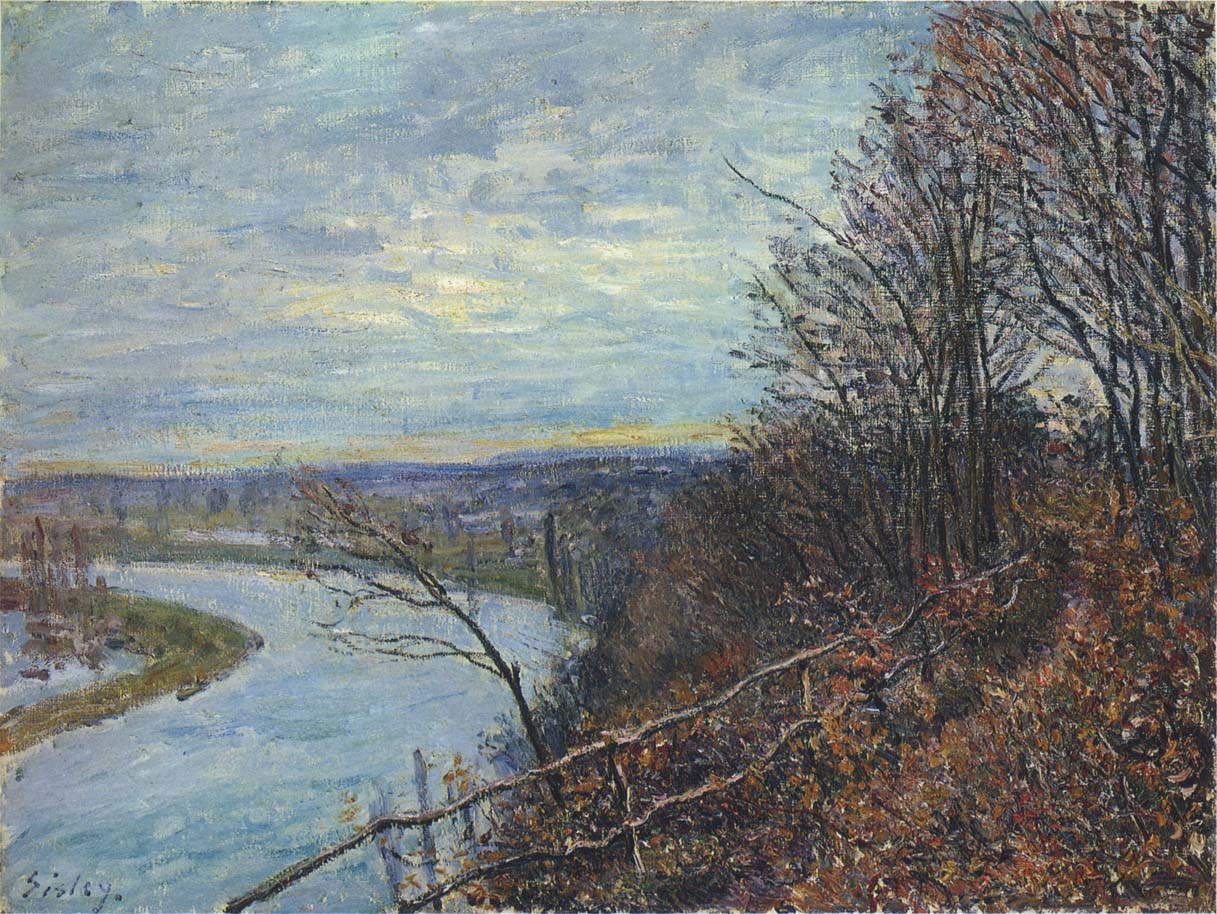The painting depicts a tranquil rural landscape at either dawn or dusk, imbued with a sense of peaceful solitude. The sky, painted with brushstrokes of blue, white, and dabs of yellow, hints at the rising or setting sun. Dominating the right half and foreground is a hill covered in brush and clusters of trees adorned with autumnal hues of brown and orange leaves, some scattered on the ground. A gently curving stream flows across the left side, bordered by grassy areas and a riverbank that extends into a pond. A wooden fence, reminiscent of days gone by, ascends the hill along a winding path threading between trees. In the distance, faint outlines of mountains are visible, enhancing the panoramic view. Additionally, near the bottom left, the artist's signature, "Cicely," is discernible. The scene evokes a serene and rural atmosphere, far removed from the hustle and bustle of urban life.